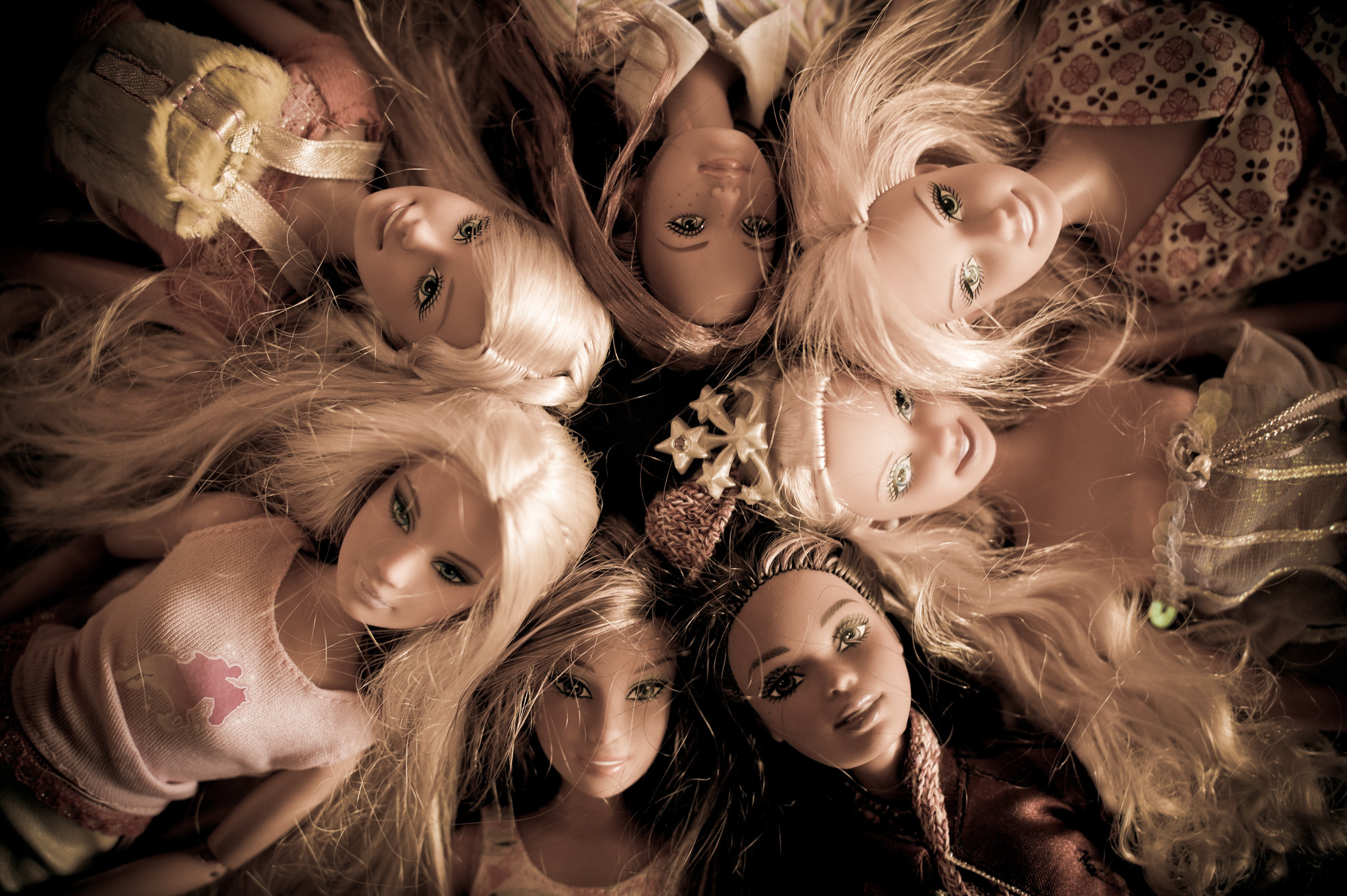The image depicts a circle of seven Barbie dolls arranged with their heads pointing inward, suggesting an aerial view where the dolls appear to be laying on their backs. This composition primarily reveals the dolls from their heads to their midsections. Among the seven dolls, most have blonde hair, with one doll having brown hair and another doll displaying a mix of dirty blonde and brown hair. The dolls, all female, exhibit a variety of facial expressions, with some smiling and others not.

They are dressed in diverse attire; predominantly dresses and tank tops. Notable details include one doll wearing a pink tank top, and another sporting a flowery shirt with brown and black floral designs. Additionally, one doll on the right side of the image is wearing a crown, while another doll appears to have a backpack worn backwards. This detailed arrangement highlights realistic eyes and facial features, contributing to an overall lifelike appearance for each doll. The image captures the dolls in a visually intricate and carefully posed circle.